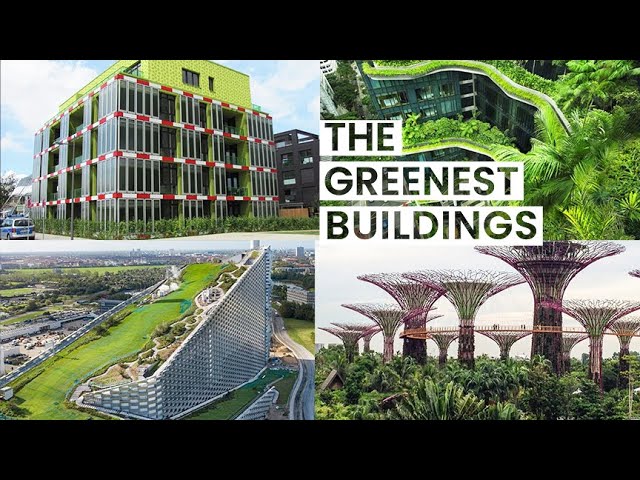This postcard-like image showcases four distinct photographs of eco-friendly buildings framed by thick black bars at the top and bottom. At the top right corner, the text "The Greenest Buildings" is prominently displayed. 

The upper left panel features a four-story building adorned with floor-to-ceiling windows and a striking red and white alternating trim around each level. The structure is surrounded by lush greenery, and the roof appears to be neon green. The building is still under construction, with visible supports.

In the upper right panel, an apartment building is surrounded by green spaces and trees, with balconies filled with verdant plant life. This viewpoint is from above, revealing areas of lush greenery and a large tree at the bottom right, underscoring the building's integration with nature.

The bottom left image depicts a tall structure with a mirrored exterior set in a meticulously manicured lawn or park. A terraced garden ascends the building's roof, highlighting its commitment to sustainability. In the background, a cityscape filled with tall buildings complements the greenery in the foreground.

The bottom right panel showcases the iconic Garden by the Bay floral towers in Singapore. These towering, modern floral structures rise majestically from the surrounding trees, resembling human-made trees with pink metal designs and interconnected walkways. A small house at the bottom emphasizes their immense scale against an overcast sky.

Together, these images collectively emphasize innovative and sustainable architecture harmoniously blended with nature.